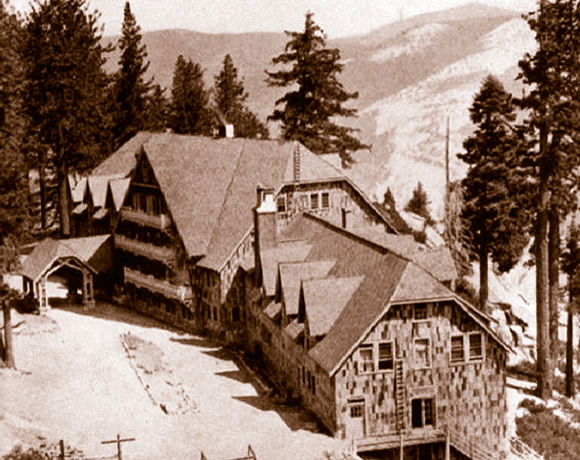This black-and-white, sepia-toned aerial photograph captures a large, historic, multi-story building that appears to be a ski resort or lodge set in a mountainous, snow-capped region. Constructed in an architectural style suggestive of the early to mid-20th century, the structure features a steep roof with uniformly distributed dormers and several levels protruding from its sides. The building is surrounded by tall, snow-topped pine trees and set against a backdrop of rugged, snow-capped mountains. 

A covered archway parkway is prominent in front of the main entrance, likely designed to protect guests from inclement weather. Various windows and balconies punctuate the building’s exterior, which seems to be clad in wooden shingles of varying hues, adding texture to the façade. Additional features include a chimney, multiple doors, and a stairway leading downhill, suggesting the building is perched on an inclined slope. The image shows power lines and possible balconies on another section of the building, indicating functional areas for guests. The cleared snowy embankments and dense tree coverage in the surrounding provide evidence that the location could be used as a ski resort. Overall, the image gives an impression of a grand yet aged mountain retreat encompassed by natural beauty.